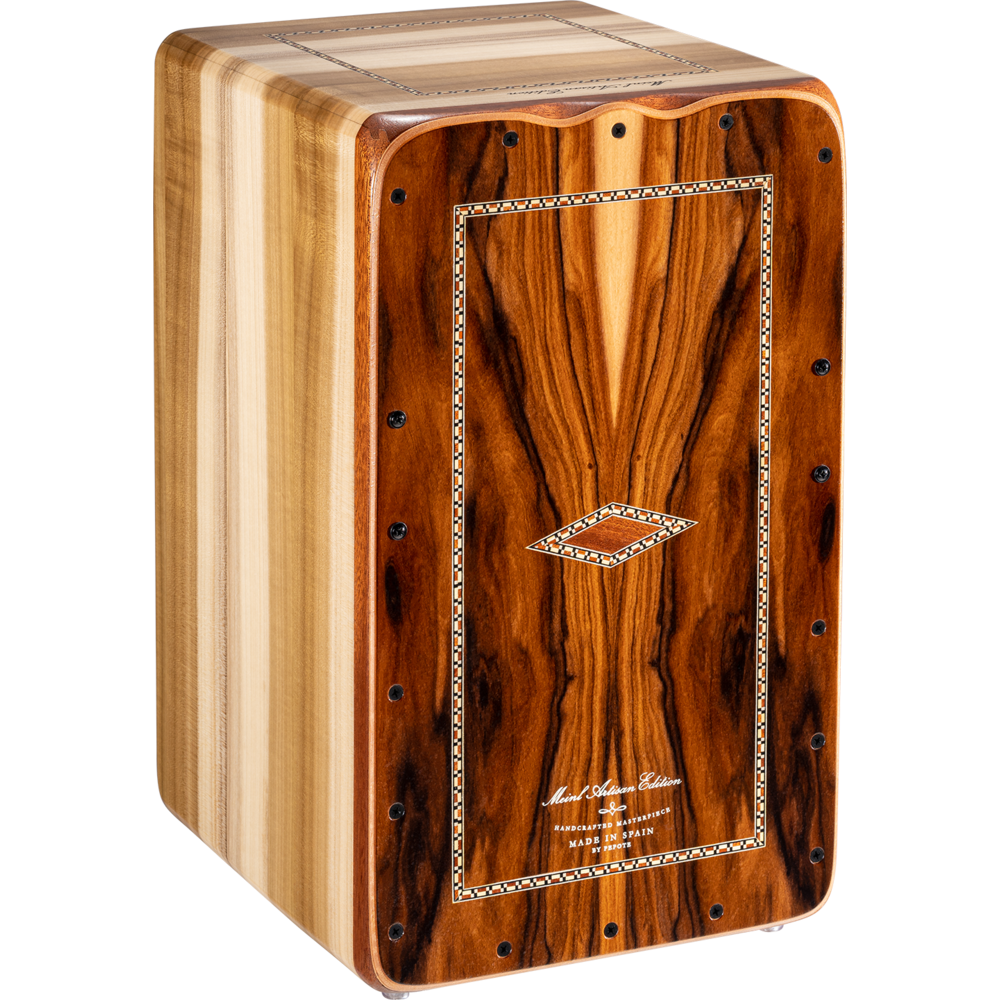This image features a rectangular wooden box, viewed at an angle with the left front corner facing the camera, showcasing both the front and left side. The box is crafted from lighter-colored wood on the sides and top, with a darker wood front. The wood appears to be natural, heavily polished, and has visible grain. Black screws are lined along the edges of the front panel, which is decorated with a notable rectangular mosaic-like design in the center. This design features a diamond shape tilted on its side, resembling a Native American pattern.

The front also displays several inscriptions: at the bottom center in small white cursive writing, though difficult to fully discern, the phrase ends with the word "edition." Below this, a stylized flower-like symbol appears, followed by some more text, which includes the phrase "handcrafted masterpiece made in Spain" in a larger font. The box has rounded corners and small rubber feet at the bottom front corners. At the very top, there is a small square decorative element that might be functional as it looks like it could open up. The background of the image is white, making it hard to tell whether the photo was taken indoors or outdoors, or during what time of day.